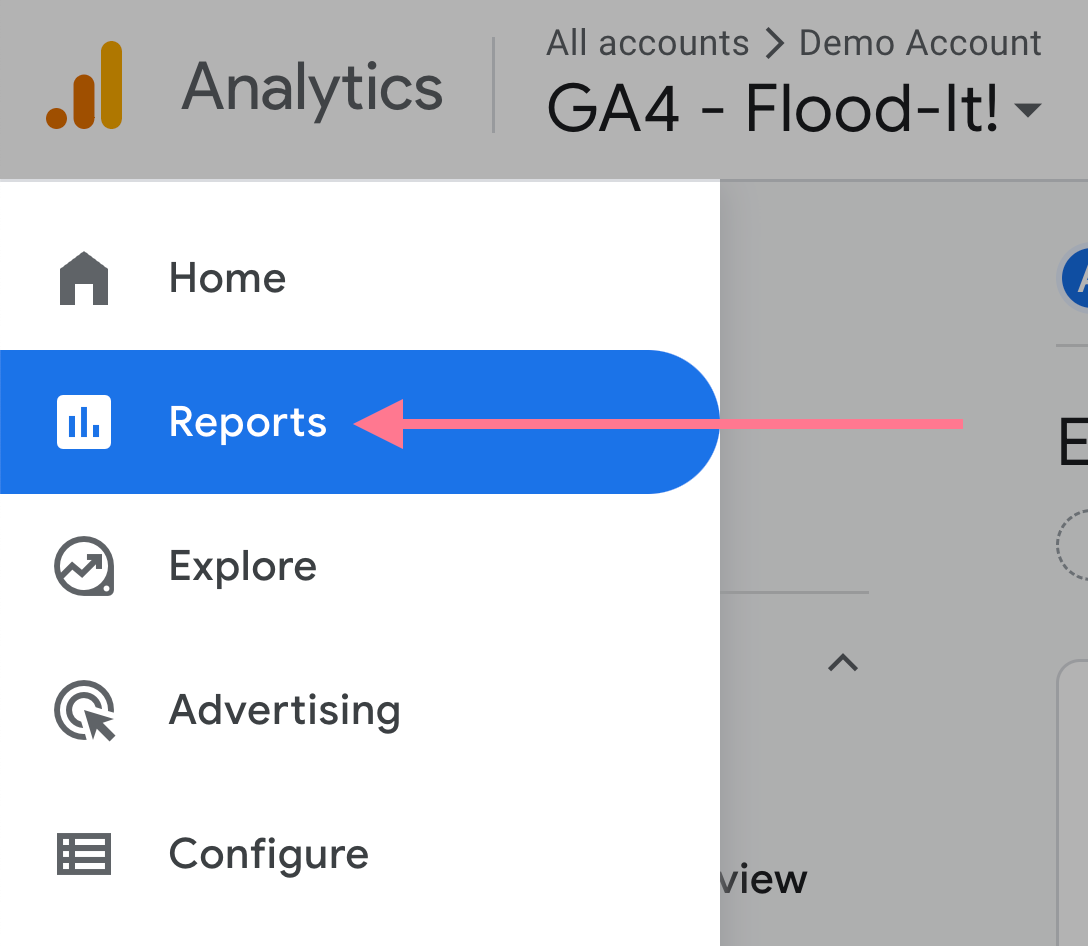In this image, we see a screenshot with a gray banner across the top. On the left side of the banner, there is a series of elements: a small orange circle, followed by an orange line, and then a gold line. To the right of this sequence is the text "analytics." Next, a gray vertical line separates this section from the rest, where smaller gray text reads "top left," "top right," "all accounts," and "demo account."

Below the banner, in large black text, the words "GA4" and "flood it" are displayed prominently. Beneath this, there is a white square featuring a navigation menu with different options and icons. At the top of this menu, "Home" is written next to a house icon. Below this, there is the word "Reports" in white text on a blue background, accompanied by a square white icon with three vertical blue lines.

Further down, "Explore" is listed in black text alongside an icon that consists of a circle with an arrow inside. Next is "Advertising," paired with a bullseye icon featuring an arrow running diagonally into it from the lower right. The last item in the menu is "Configure."